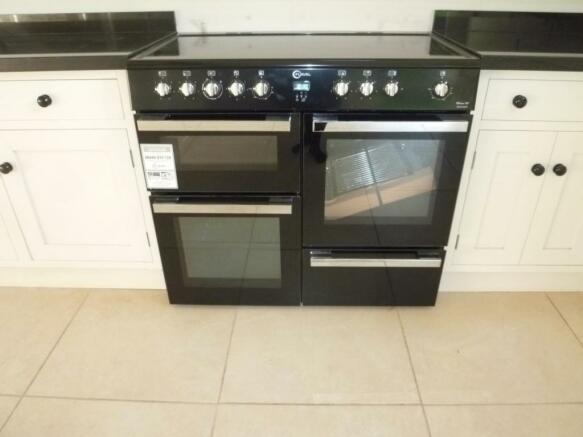The image captures a stylish kitchen featuring a prominently positioned black kitchen range with an impressive array of features. Dominating the center of the scene, the range appears to be a double or triple oven configuration, wider than typical ovens, with distinct sections. The left side showcases a dual-chamber setup, with a smaller upper oven and a larger one beneath it. To its right, there's a standard large oven door, complemented by a storage compartment below. 

The range is adorned with a total of nine knobs, primarily in white with silver chrome accents, distributed across the unit. Black countertops, possibly granite, flank the range on both sides, bordered by white cabinets. The kitchen floor features large tan tiles, adding to the room’s modern appeal. This new, possibly freshly installed setup hints at a chic and functional kitchen space ready to be utilized.